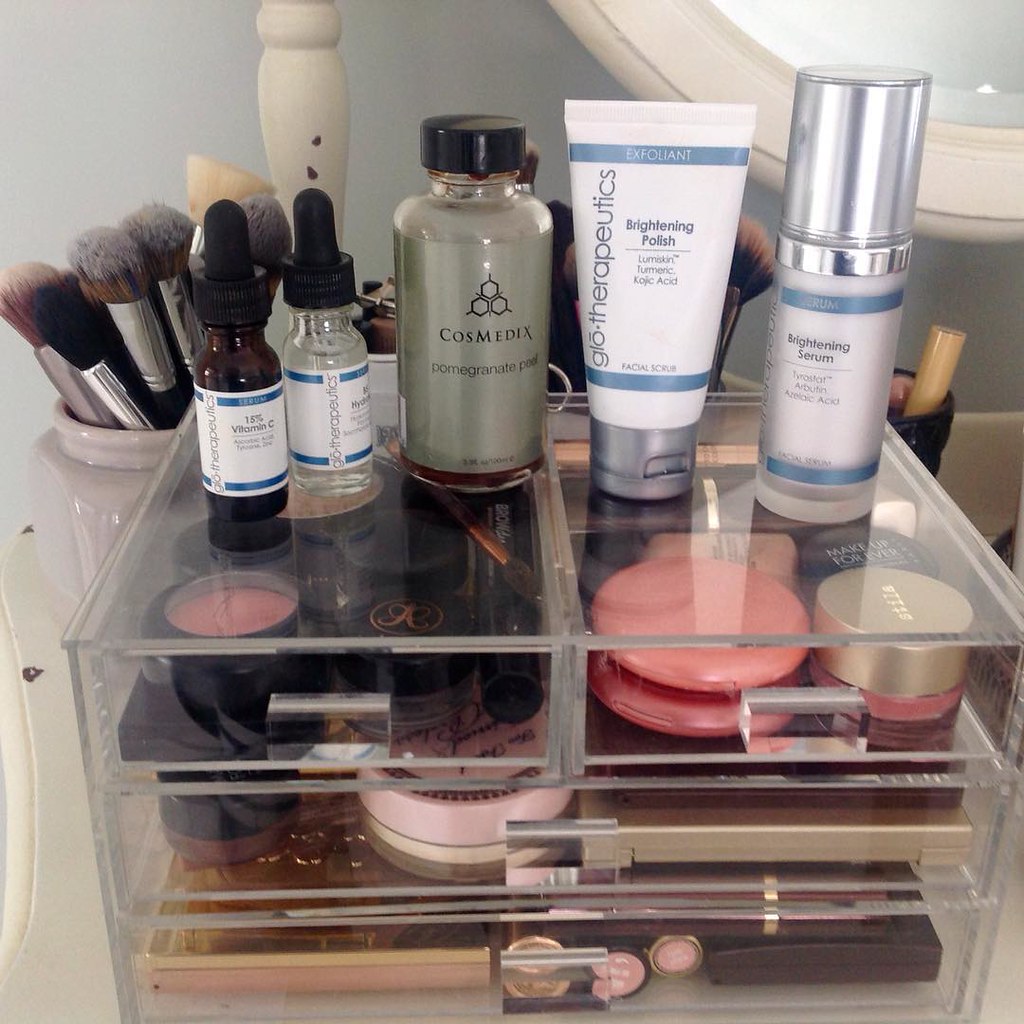This image features a transparent makeup organizer with four distinct compartments. The organizer is positioned on a white countertop, likely located in a bathroom, as evidenced by the mirror hanging on the light blue wall behind it. The upper section of the organizer consists of two side-by-side compartments. The left compartment holds various makeup items, including blushes and lip glosses, while the right compartment contains skincare products like eye creams and a couple of pink compacts. Beneath these, the middle compartment, though partially obscured, appears to store an eyeshadow palette. The bottom compartment includes a gold eyeshadow palette and several maroon-colored lipsticks.